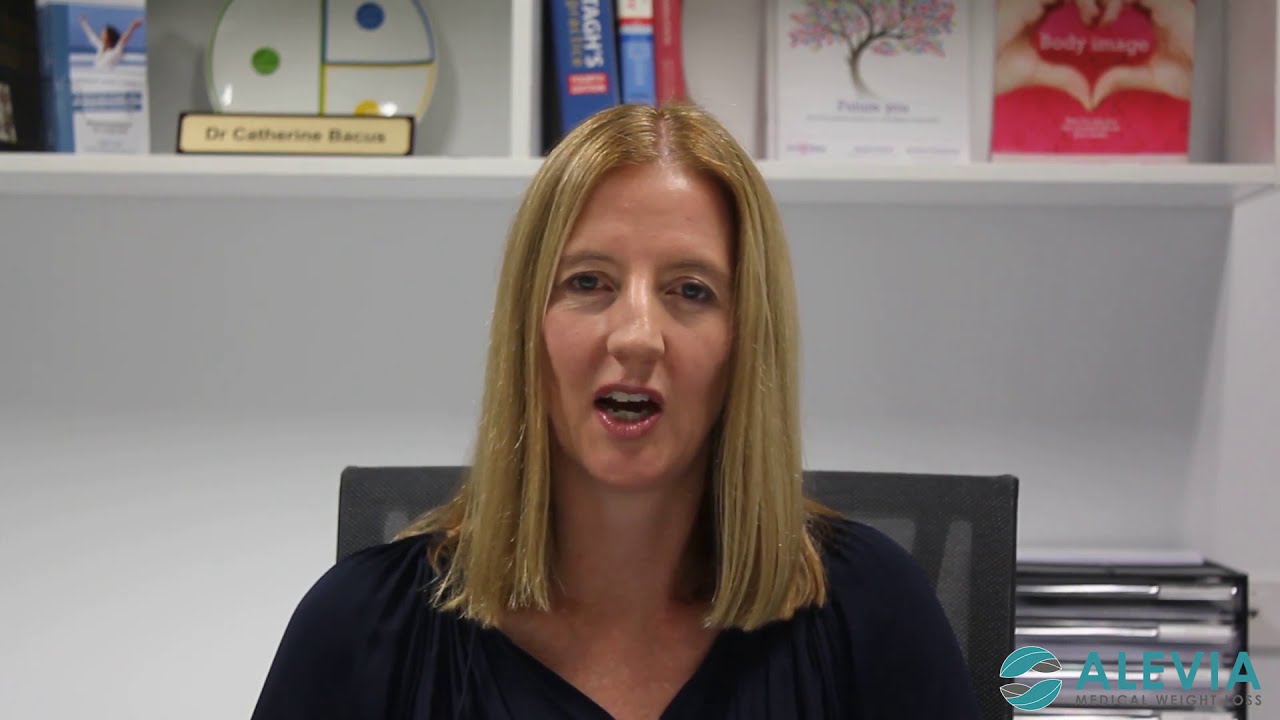The image depicts a woman sitting in a chair, captured from the chest up, likely mid-sentence. She is dressed in a business-professional black V-neck shirt, and has straight, shoulder-length, reddish-blonde hair. The main background features a white wall and a slightly blurred bookshelf behind her, filled with books, including one with a tree on its cover and another showing hands making a heart symbol. On the top left of the bookshelf is a small nameplate that reads "Dr. Catherine," though the last name is difficult to discern but might be "Bacon." Additionally, a logo at the bottom right states, "Olivia, Medical Weight Loss, Dr. Catherine Bacon," suggesting the setting could be a medical facility or doctor's office. The overall scene is framed indoors with neutral colors, predominantly white, and elements of gray, black, yellow, light blue, red, blue, and green.